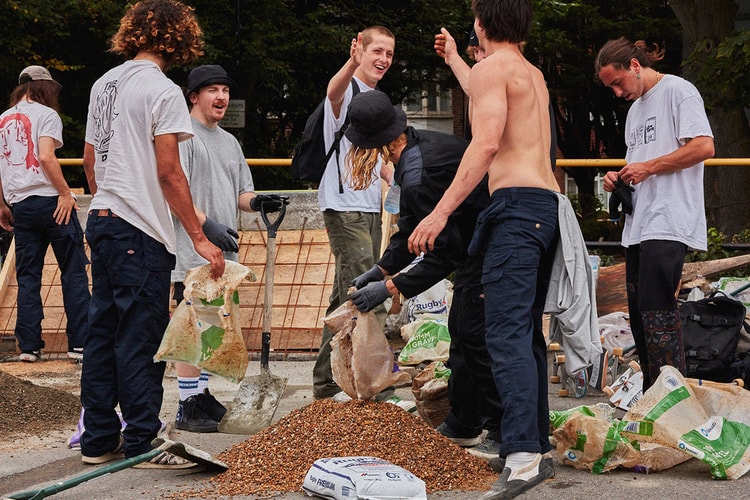In the colored photograph with a dark background, there is a group of seven young men engaged in work that involves a large pile of brown gravel, surrounded by empty bags. On the far left, a man wearing a white shirt and dark pants faces away from the camera. Nearby, two men are positioned: one in blue pants and a white t-shirt holding a bag, and another in a gray shirt with a black hat, black shoes, white tube socks, and a shovel. Central to the image is the gravel pile, with additional participants around it. One individual in green pants and a white shirt is extending his right hand, appearing to high-five a shirtless man in blue pants who has a gray shirt tucked into his waistband. Adjacent to them is a man in a derby-style hat, gray gloves, and black attire. On the right side, a man with brown hair in a ponytail, dressed in a gray t-shirt and black pants, is seen putting on gloves. The scene suggests they are preparing sandbags or shaping a pit, evident from the shovels and scattered empty bags.